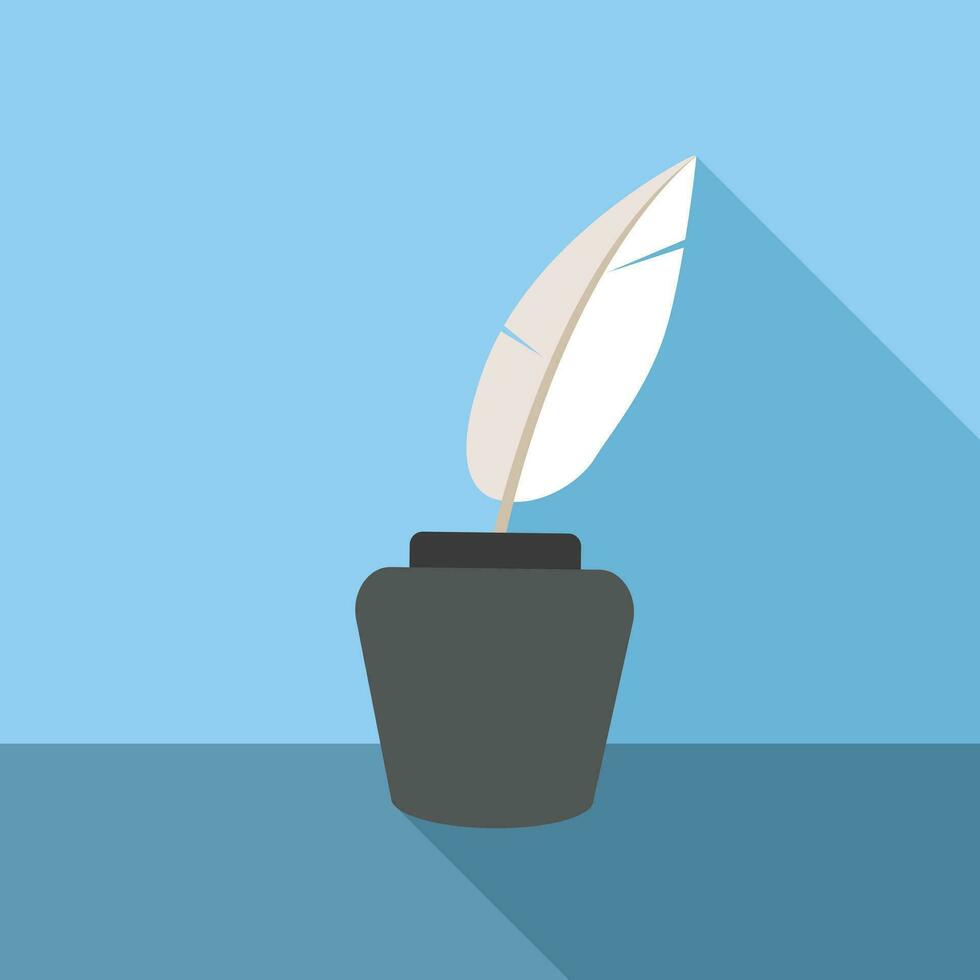This digital clip art image features a simple yet striking composition set against a two-tone blue background. The floor, rendered in a darker blue, contrasts with the lighter blue back wall, creating a spatial context. Positioned centrally in the image is a black ink pot, erroneously referred to as a vase by some, which supports a single large feather. This feather is distinctively bi-colored—pinkish on the left and white on the right—accentuated by a dark pink quill spine running up its center. The feather's elegant form, showcased by subtle splits on either side, casts a lighter blue shadow to the right, suggesting light source from the left. Overall, the image offers a visually appealing and cartoonish portrayal of an ink pot and feather.